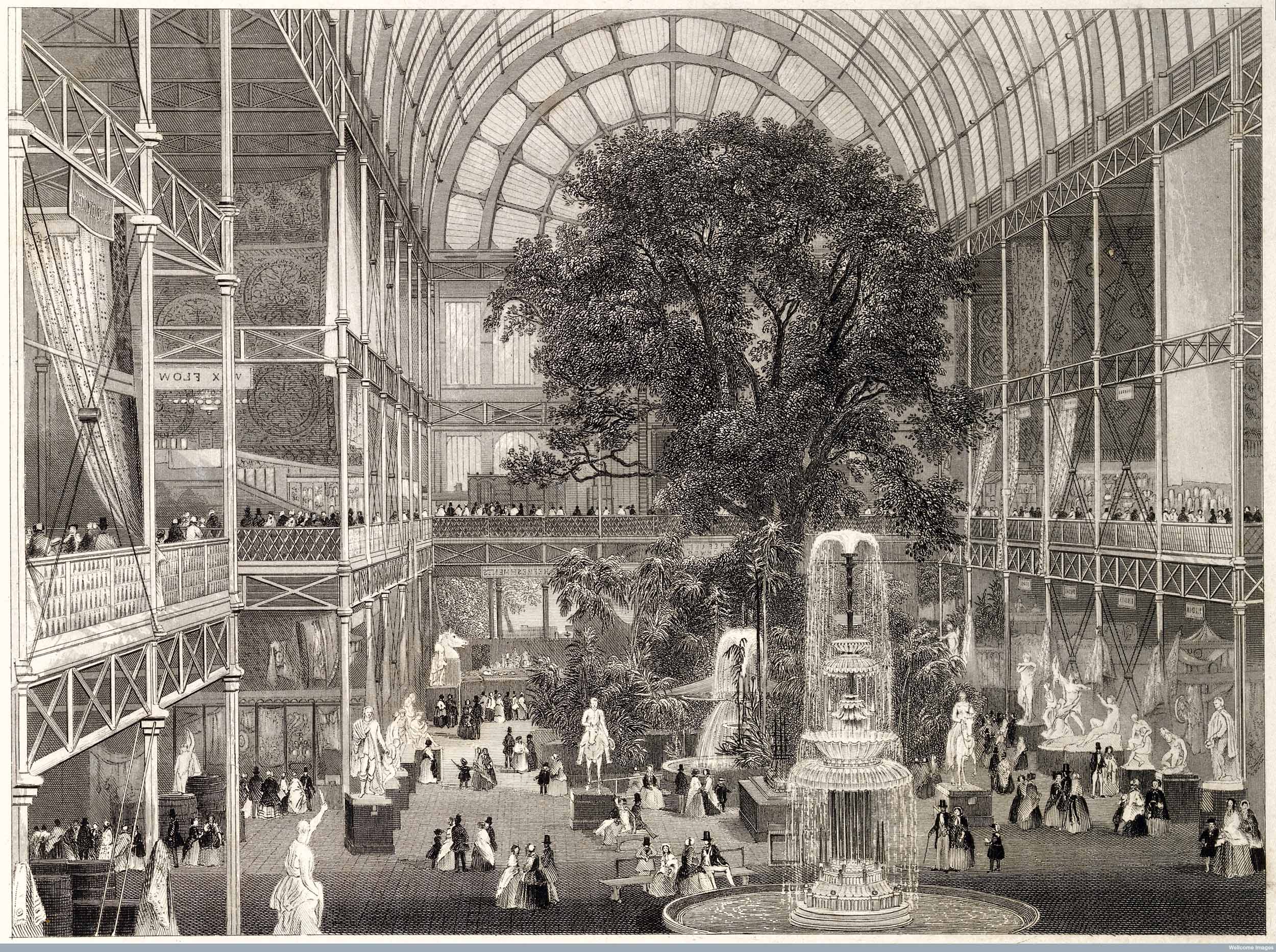The image depicts the interior of a grand, three-story atrium in a hand-drawn, black-and-white style, likely from the Victorian period. The space is expansive, with large glass panels in the domed ceiling allowing natural light to flood in. At the center of the atrium stands a colossal tree, reaching the full height of the three floors. Surrounding the tree are two ornate, multi-tiered water fountains. On the ground level, statues of various figures line the atrium walls. The scene is bustling with people dressed in period attire—women in bell-shaped dresses and men in top hats and suits, some carrying canes. On the second floor, spectators observe the busy scene below, while the third floor appears vacant aside from some bars or structural elements. The detailed illustration captures a lively, historic ambiance akin to that of an old-fashioned mall or a museum atrium.